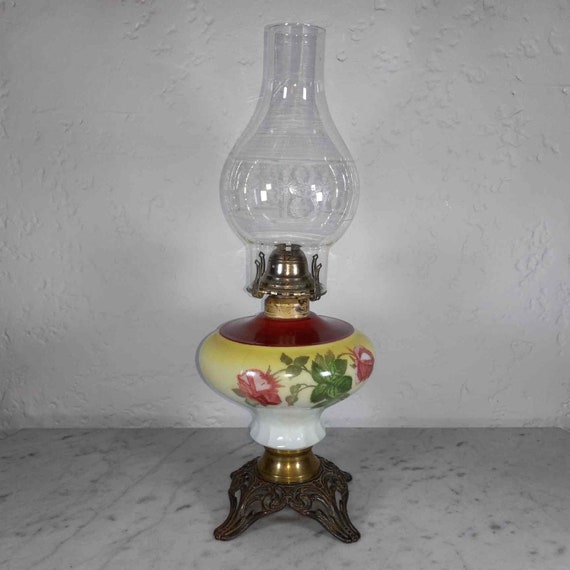The photograph depicts an antique kerosene lantern situated on a white floor against a white wall. This intricate lamp features a transparent, circular glass dome at the top and sits on a dark brown tripod base with brassy neck accents. The lamp's bulging container is a circular piece of yellow pottery, adorned with detailed floral designs, showcasing red flowers and green leaves. Below this, there's a white porcelain section bordered in yellow, contributing to the lamp's ornate and vintage appearance. The antique nature of the lamp is highlighted by its old-fashioned glass dome and intricate metal legs, exemplifying a classic style of lighting fixtures.